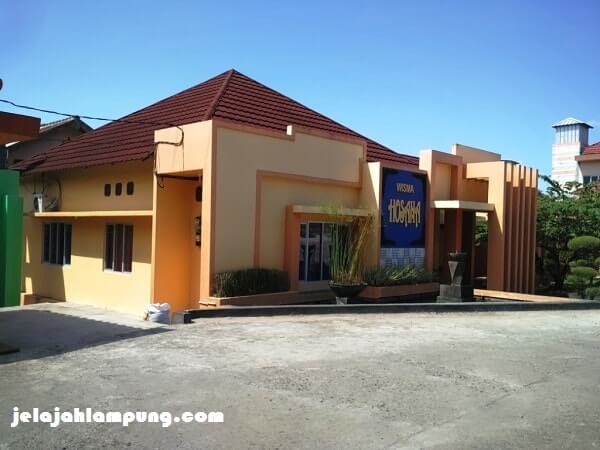The image depicts a building with a slanted brown or terracotta roof and walls that are a mix of beige, yellow, or peach stucco. The windows are black, casting heavy shadows on the left side. There is a grey concrete ground in front of the building, which shows signs of aging with white tinges. On the left side, there is a shelf near the building, a small trash bag on the ground, and what appears to be a green wall which might be a fence or gate. 

A blue and black sign with yellow lettering, possibly in a different language, is mounted on the right side of the building, accompanied by light and dark blue squares underneath it. In front of the sign and the building entrance are patches of shrubbery. The scene also includes a paved parking area. In the background, larger buildings are visible against a bright blue sky. Additionally, there is text at the bottom left of the image that reads "jaylajalampung.com."